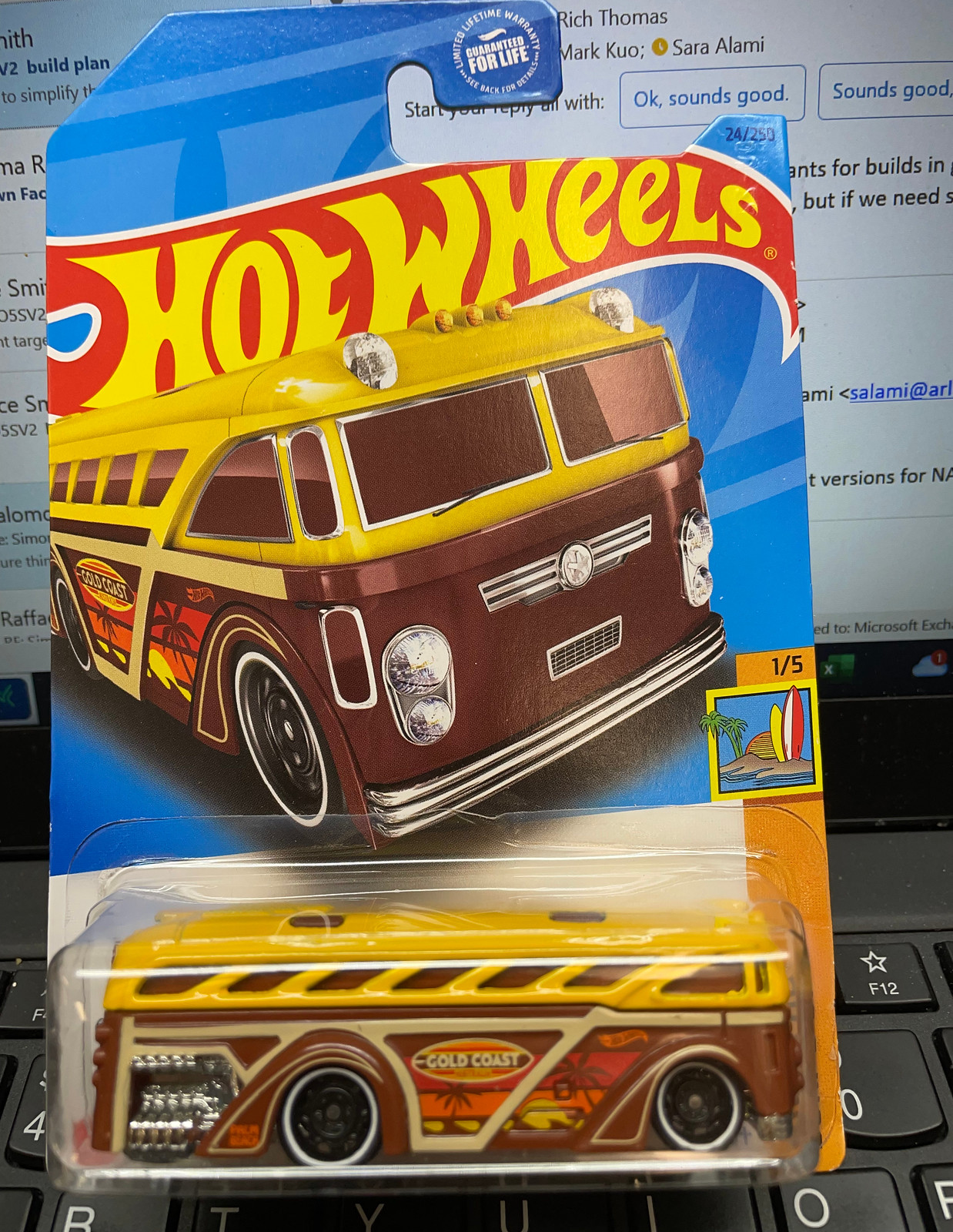The image features a straight-on view of an unopened Hot Wheels toy car still in its packaging. The toy car is a distinctive vehicle with a vintage design, resembling a VW bus but modified to look more like a roadster. The car has a brown bottom and a yellow top, adorned with a "Gold Coast" logo on a surfboard emblem on its side, accented by graphics of palm trees and a sunset. It is fitted with black wheels featuring a white line around them, and a shiny metallic engine detail is visible at the back.

The Hot Wheels car is encased in a clear, rectangular plastic bubble, which is affixed to a piece of cardboard. The cardboard backing prominently displays the Hot Wheels logo, rendered in yellow against a red flame banner across the top. It also includes a detailed graphic of the car. This packaging sits on top of a black computer keyboard with white lettering, partially obscuring the keys. 

In the background, a computer monitor with a black plastic rim is visible, displaying some form of online interaction, such as a forum or email program. The entire scene effectively captures the vibrant and nostalgic essence of the Hot Wheels brand, set against a backdrop of everyday digital life.